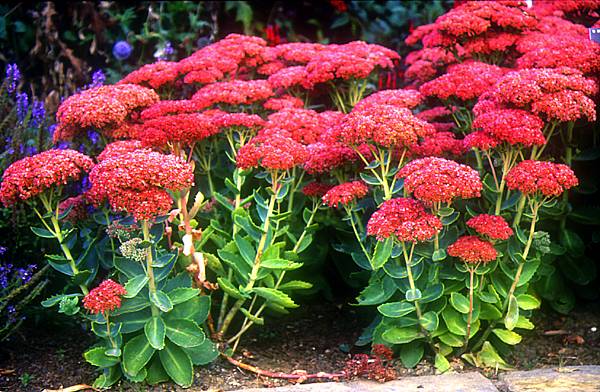This detailed photograph depicts a vibrant garden scene, horizontally oriented with no text overlay. In the well-lit foreground, vivid red multifloral heads burst atop succulent-like green stems and short, thick leaves, reminiscent of milkweed or possibly a cultivar of hydrangeas. The fluffy red flowers are notable for their width and numerous small petals, sprouting robustly from healthy, waxy green foliage. Among these, one red flower lies wilted on the stone pavers below, which are interspersed with patches of dirt suggestive of a pathway in a private or public garden.

To the left in the background, a cluster of tall, narrow purplish-blue flowers, possibly lavender, stand out against darker green plants and blurred greenery, adding depth and variety to the composition. This backdrop of generalized foliage creates a natural setting that emphasizes the garden's lushness and the plants' vibrant health. The interplay of light and shadow enhances the beauty of the scene, giving the photograph a realistic and inviting feel.